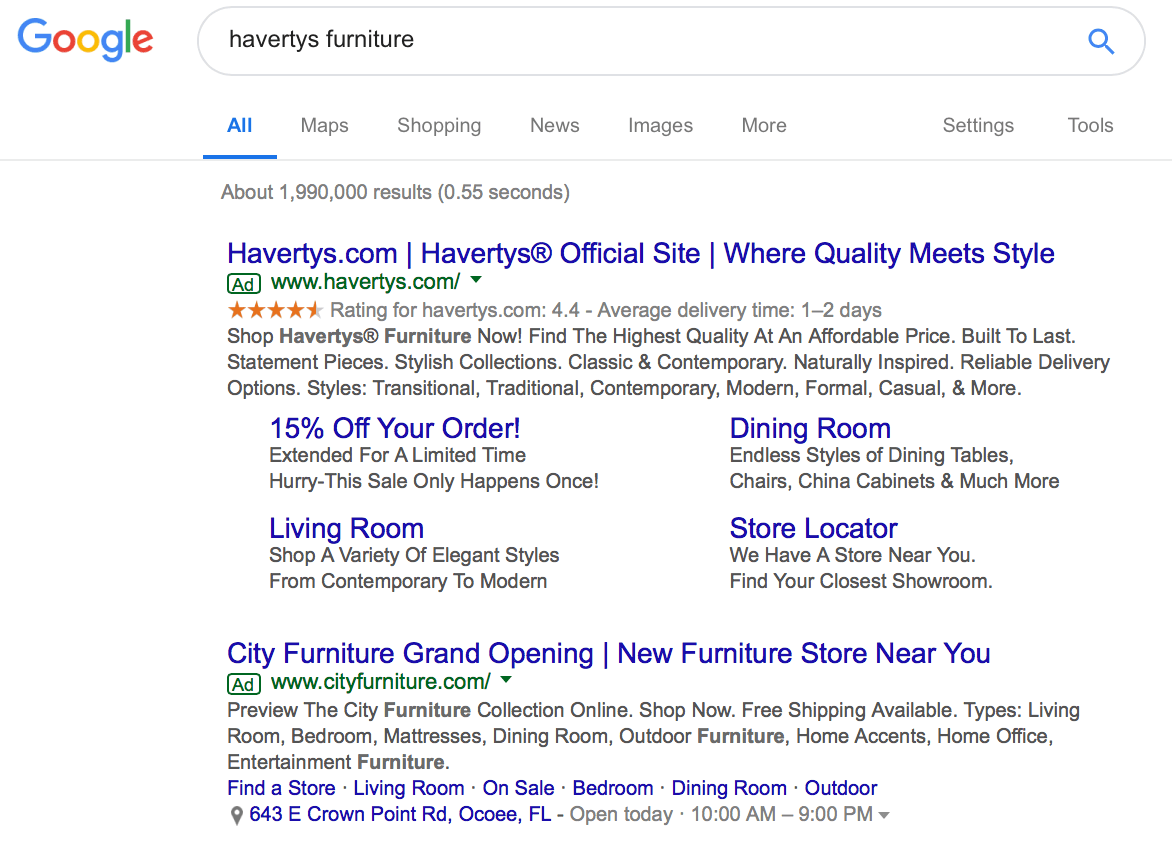This image features a Google search results page where the search query is "Haverty's Furniture". The page indicates approximately 1,999,000 results that were retrieved in 0.55 seconds. The first search result displays the official website link "Haverty's.com" in blue, accompanied by the tagline "Haverty's Official Site - Where Quality Meets Style". Below this, the URL "www.haverty.com" is shown in green, and the site boasts a 4.4-star rating.

The site promises an average delivery time of 1-2 days. A call-to-action below encourages users to "Shop Haverty's Furniture Now" and highlights that they offer high-quality, affordable furniture that is built to last. The collection features a range of statement pieces encompassing both classic and contemporary styles. Customers are assured of reliable delivery options and can browse a variety of styles including traditional, contemporary, modern, formal, and casual.

Additionally, there is a promotional note indicating a 15% discount on orders that is extended for a limited time, urging customers to take advantage of the sale quickly. The promotion emphasizes that such deals happen only once, and specifically mentions a variety of elegant living room styles available, from contemporary to modern.